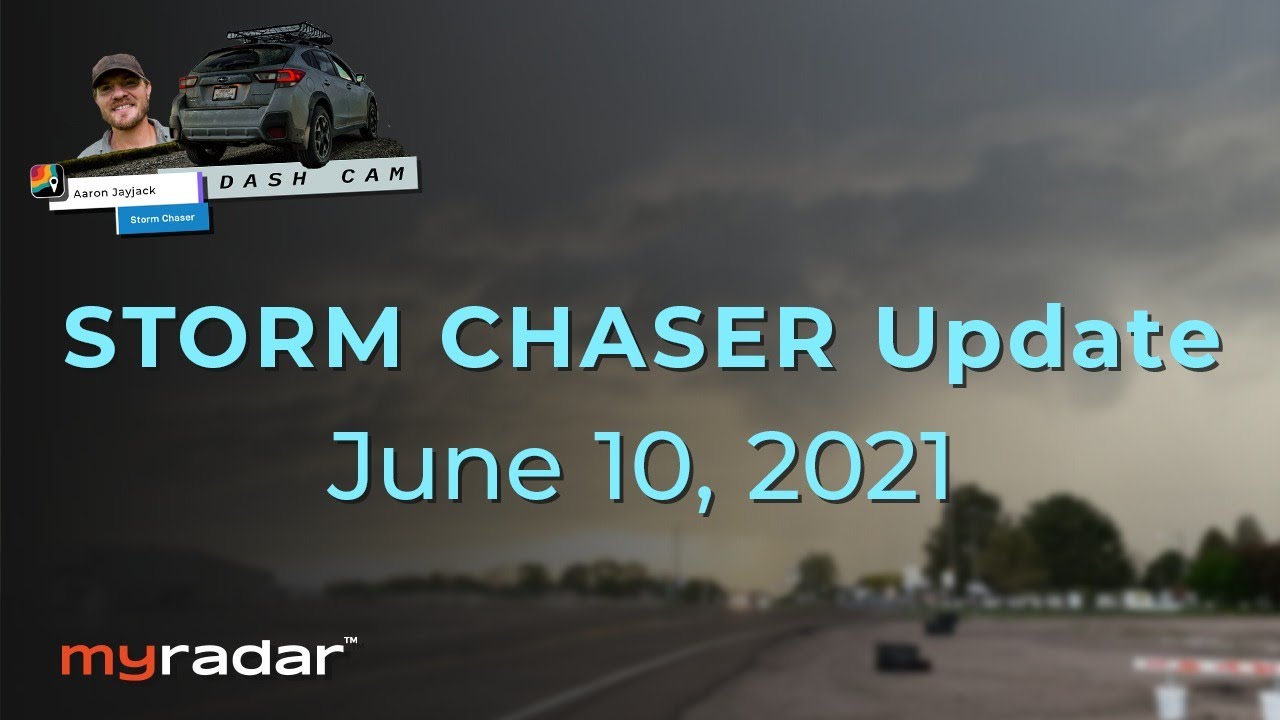The image seems to be a promotional ad for an app called "MyRadar," likely related to weather tracking. The name "MyRadar" is displayed in the bottom left corner with "My" in red and "Radar" in white, all in lowercase letters. Dominating the upper left corner is a photograph of Aaron Jayjack, a well-known storm chaser, recognizable by his ball cap, beard, and mustache. Next to him is a car equipped with a dash cam, underscoring his role in chasing storms. Centrally placed in the image, in light blue writing, is the phrase "Storm Chaser Update," followed by the date "June 10th, 2021." The background of the image is quite dramatic, showcasing dark, menacing clouds and hints of tornadoes, with unique trees and a tree line visible, highlighting the severe weather that Aaron is documenting.